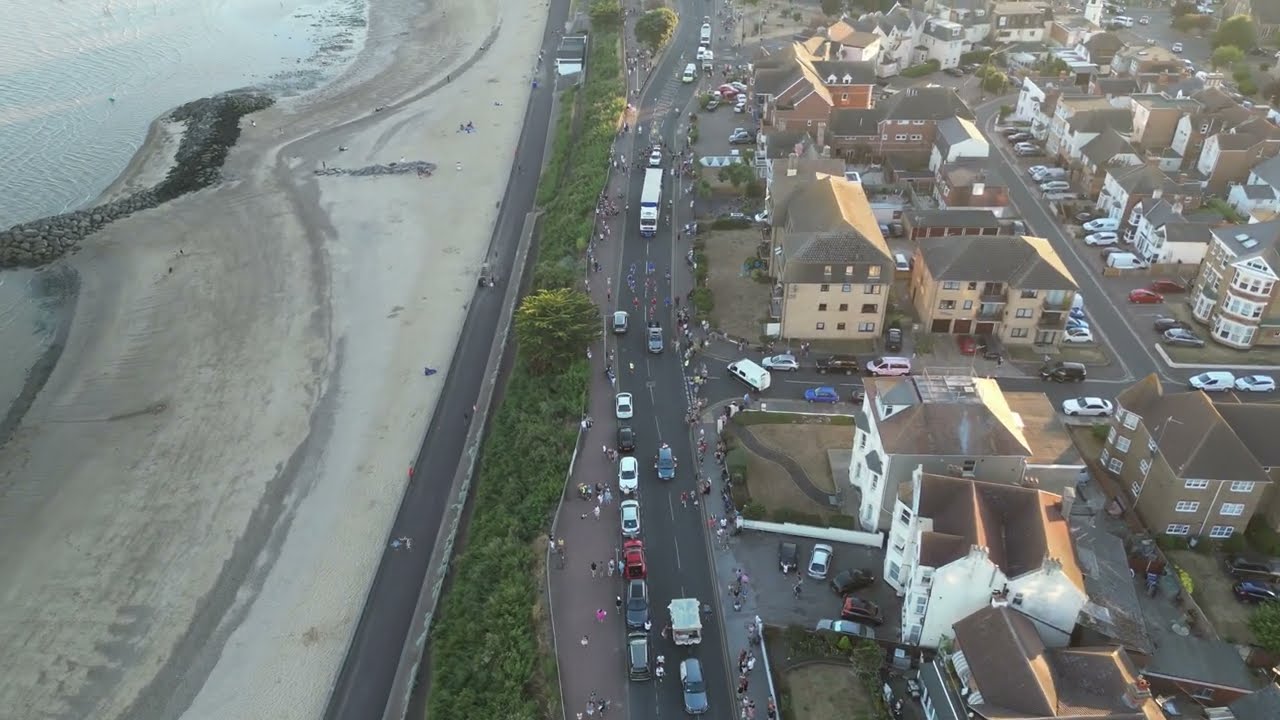The aerial image depicts a small coastal town in the late afternoon, bathed in natural light. Positioned on the left side of the frame, a body of water, likely part of a lake or beach, stretches parallel to a sandy shoreline, slightly cut off from view. Adjacent to the shore is a walking path lined with green grass and trees, adding a touch of natural verdancy to the scene. Moving further to the right, a multi-lane highway runs vertically through the center of the image from top to bottom, serving as a central artery for the town.

On the far right, a residential area comprising mainly two to three-story homes and apartment buildings sprawls across the landscape. These buildings range in color from off-white and beige to brown and red, contributing to a diverse yet harmonious streetscape. The residential zone appears devoid of commercial establishments and is teeming with cars and pedestrians, giving life to the scene. The image, free from any readable text or numbers, showcases a vibrant community set against the picturesque backdrop of a tranquil shoreline and verdant surroundings.